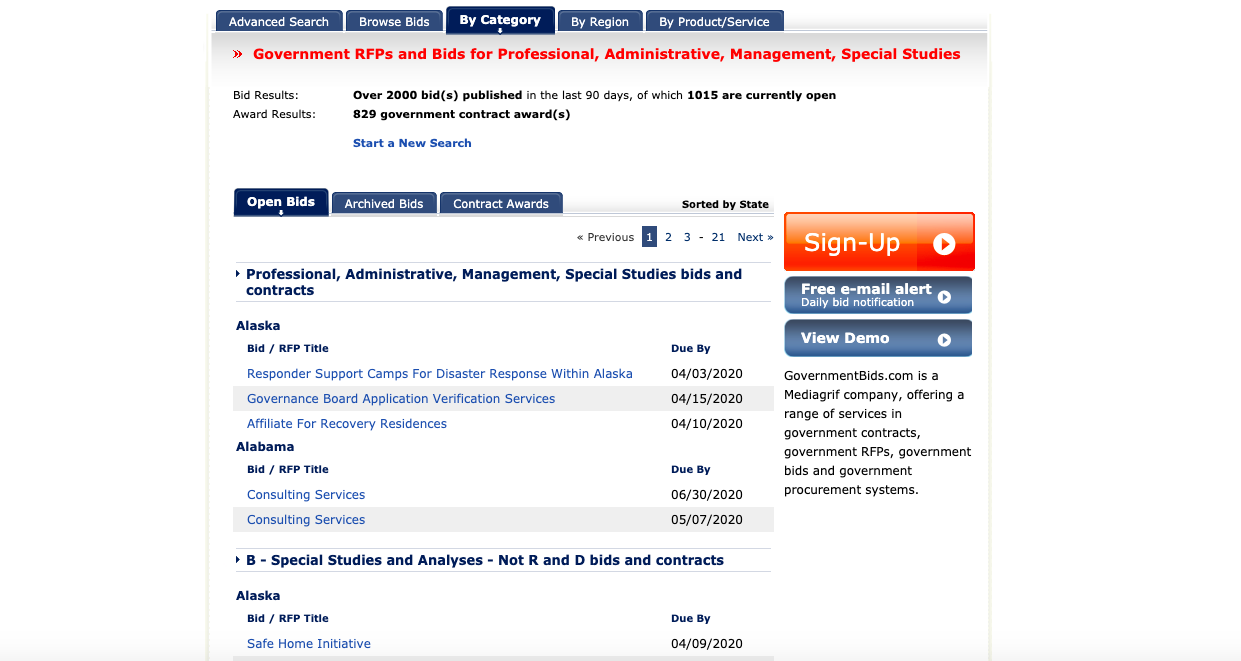The image is a screenshot of a government procurement website displaying various features and information. At the top of the page are several navigation tabs in blue with white font: "Advanced Search," "Browse Bids," "By Category," "Region," and "By Product Service." The "By Category" tab, currently selected, is highlighted in a slightly darker blue.

Below the tabs, in red font, is the heading "Government RFPs and Bids for Professional Administrative Management Special Studies." In black font underneath, it states "Bid Results, over 2,000 bids published in the last 90 days, of which 1,015 are currently open," and "Award results, 829 government contract awards." 

In blue font, there is a link to "Start a New Search." Below this, additional navigational tabs for "Open Bids," "Archived Bids," and "Contract Awards" appear, with "Open Bids" highlighted in a darker shade of blue, indicating the current section.

The content is sorted by state, indicated in black font, and includes a sidebar with action buttons. A gradient orange-to-red rectangular button labeled "Sign Up" features a play button arrow on the right side. Below it, two gradient blue rectangular buttons offer options for "Free Email Alert, Daily Bid Notification," and "View Demo."

At the bottom left, a note states, "GovernmentBids.com is a MediaGriff company offering a range of services in the government contracts, government RFPs, government bids, and government procurement systems." Adjacent to this note, the main content outlines sections for "Professional Administrative Management, Special Studies, Bids, and Contracts" and "Special Studies and Analyses (non-R&D), Bids, and Contracts," listing some from states like Alaska and Alabama. The main content columns display "Bid and RFP Titles" and "Due By" dates.